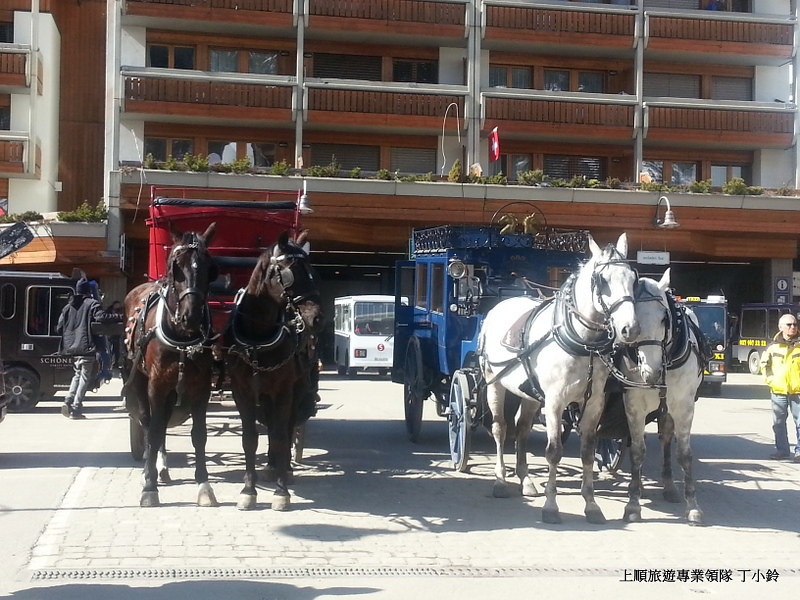This horizontal, rectangular color photograph captures a lively street scene in an urban environment. At the center, two pairs of horses draw carriages: the left pair, brownish-black, pulls a red carriage, while the right pair, white or whitish-gray, pulls a blue carriage. The horses stand on a tar-red road with various vehicles around them, including a small white van and two black cars on the right side, one of which has yellow writing.

In the background, a high-rise apartment building stands prominently, characterized by its wooden facade and tightly spaced windows, which provide privacy for each unit. One resident, wearing a white vest, is visible looking out from a lower window. On the right, another apartment building adds depth to the scene.

A man in a yellow jacket and blue jeans, possibly of Asian descent, stands near the carriages. Another man, dressed in all black with grey jeans and a black beanie, stands next to one of the black cars on the left. Chinese characters are inscribed in the lower right-hand corner of the image, suggesting a location in China. The street is bustling with urban life set against the multifaceted backdrop of apartment balconies and shaded windows.